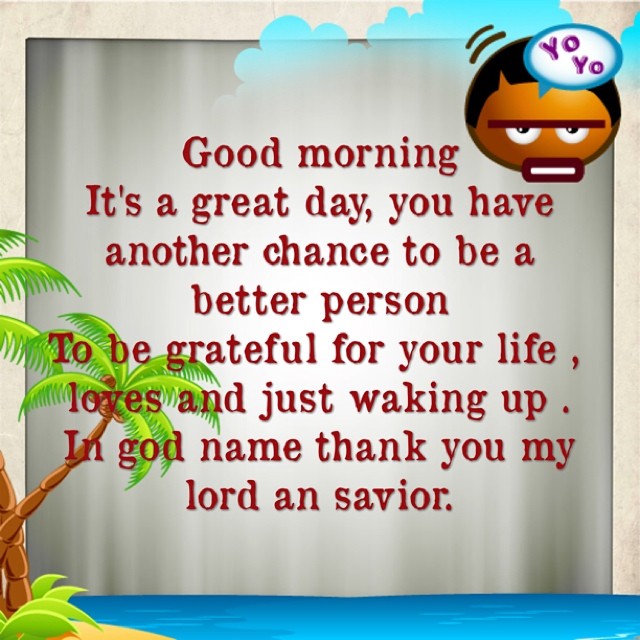The image is a digitally created, cartoony, inspirational poster set against a predominantly gray background with light gray borders. It features a tropical theme on the bottom left, where a small island with palm trees and blue water is depicted. Towards the top right, there is a cartoon emoji with brown skin, short black hair, and a frustrated expression, characterized by flat eyebrows and an open horizontal mouth. The emoji has a speech bubble that says "yo-yo" in blue and purple text. In the center of the image, in prominent brown text, is an inspirational message that reads: "Good morning, it's a great day. You have another chance to be a better person, to be grateful for your life, loves, and just waking up. In God's name, thank you, my Lord and Savior." The background also features subtle elements like a painted blue cloud towards the top, adding to the whimsical and motivational feel of the poster.